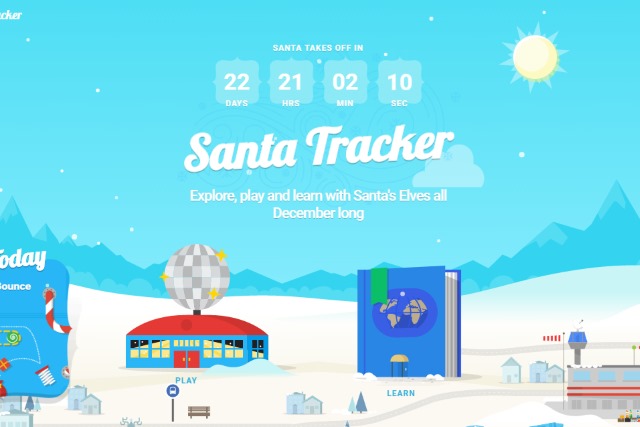**Caption:**

The screenshot showcases a vibrant, interactive Santa Tracker website designed for advent festivities. Dominating the center, the phrase "Santa Takes Off In" is prominently displayed, accompanied by a countdown timer showing 22 days, 21 hours, 2 minutes, and 10 seconds, heightening the anticipation of Santa's journey. The background is a light sky blue, featuring a whimsical polar city scene adorned with snowy landscapes and festive elements.

At the center is a playful white cursive "Santa Tracker" logo, overlaying a subtle watermark or hidden image, possibly a butterfly or floral design. The website invites users to "Explore, play, and learn with Santa's elves all December long," encapsulating the interactive spirit of the season.

The bottom third of the screen brings the polar cityscape to life, with detailed depictions:
- On the left, a billboard sign with a candy cane striped pole emphasizes today's activities.
- Moving right, a festive arena or stadium, marked with a large disco ball, invites visitors to "play."
- In front of the arena, a bus stop adds to the city scene's realism.
- Further right, a giant blue book with a green bookmark and a yellow-canopied door symbolizes opportunities to "learn." 
- Lastly, the bottom right corner houses an airport, identifiable by its air traffic control tower and windsock, hinting at Santa's upcoming departure.

Above the snowy terrain, faint, darker blue mountains frame the backdrop, while the full sun beams from the top right corner, casting a cheerful light across the scene. In the upper left corner, the "Santa Tracker" text is partially visible, teasing the entirety of the joyous interface.